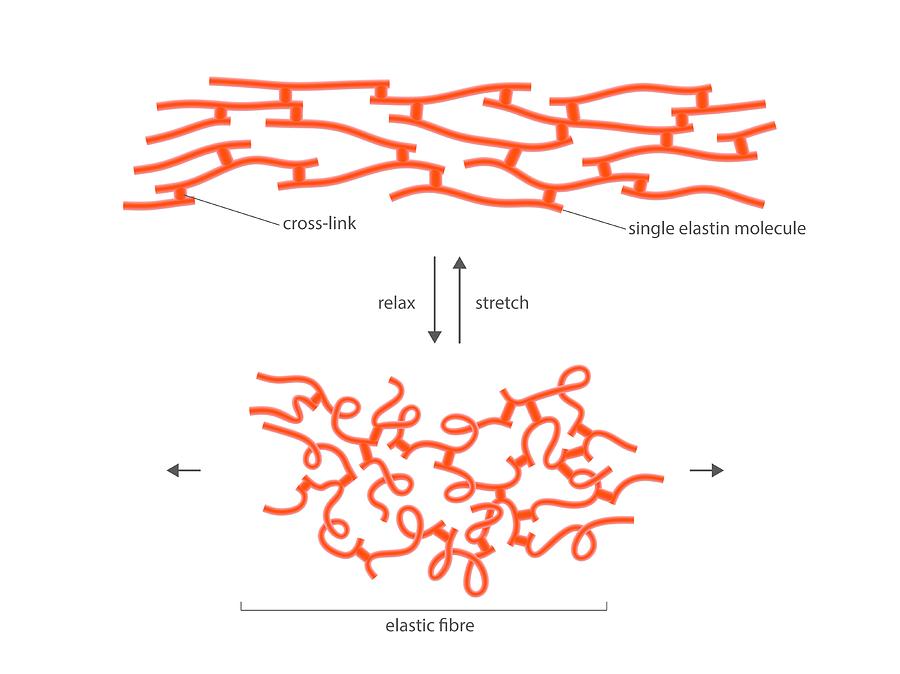The scientific diagram illustrates the structure and behavior of elastin fibers. At the top, thin, red, worm-like shapes, each with small circles at their ends, form an interlaced, bright orange lattice structure. The lower left part of the diagram highlights one of these circles, labeling it as a "cross-link." On the lower right, it points to one of the lines, identifying it as a "single elastin molecule." Below this section, the diagram includes two directional labels: "relax," with a downward arrow, and "stretch," with an upward arrow. At the very bottom, a detailed illustration shows the elastin molecule coiled or scrunched together, with arrows pointing left and right, indicating the flexible nature of the structure. This part is labeled as "elastic fiber." Overall, the diagram provides a comprehensive visual representation of elastin's molecular makeup and its elastic properties.